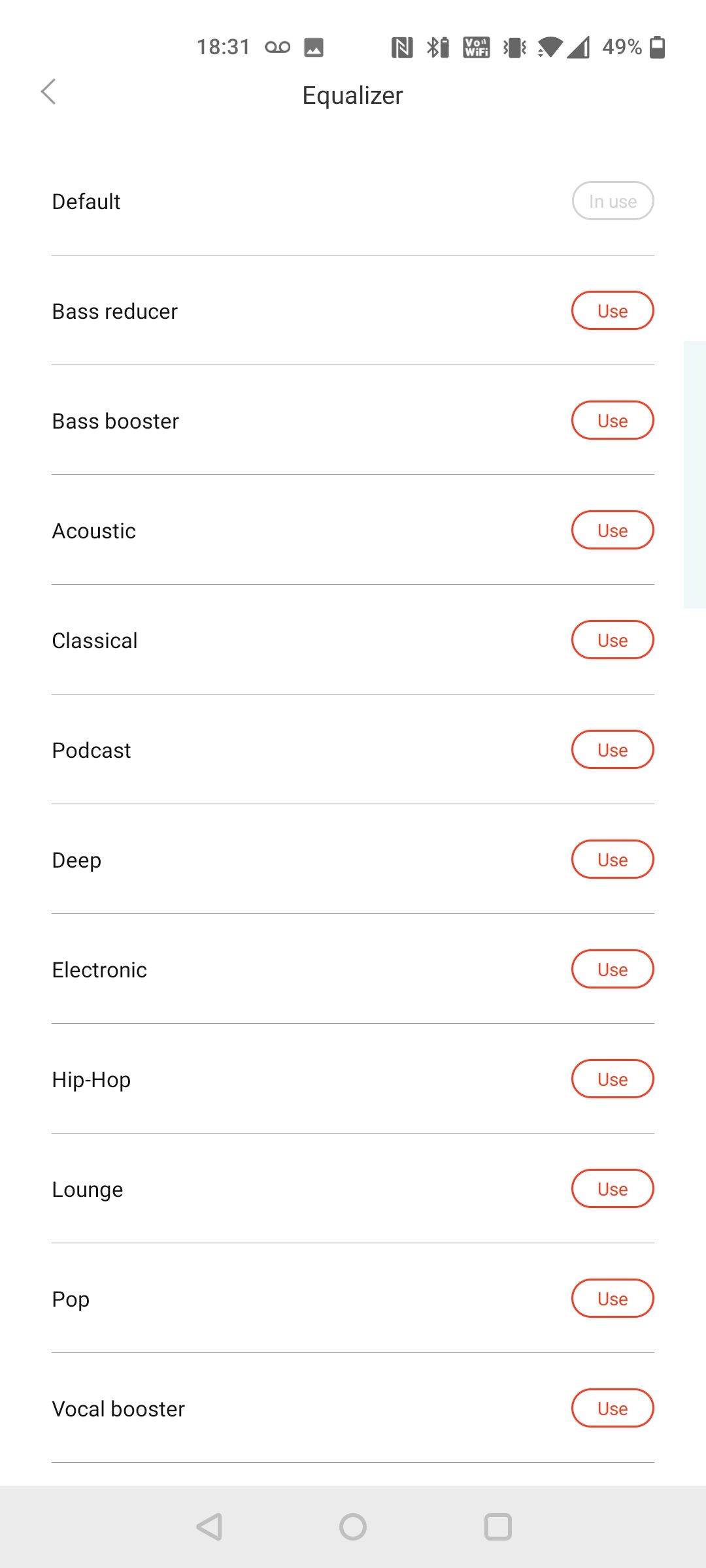In this image, we have a screenshot of a cell phone display set against a clean, solid white background. The top left corner of the screen shows the time "18:31" next to a small icon representing a gallery. Directly to the right of this icon are additional status icons: a box with what appears to be the letter 'N' inside, the battery icon displaying 49% charge, and the Wi-Fi signal indicator.

Central to the image is the word "Equalizer," prominently displayed. Below it, there's a list of equalizer settings, each one aligned to the left with a corresponding "use" button on the right. The list is as follows from top to bottom:

- Default
- Bass Reducer
- Bass Booster
- Acoustic
- Classical
- Podcast
- Deep
- Electronic
- Hip Hop
- Lounge
- Pop
- Vocal Booster

Each of these options provides a different audio preset, allowing users to customize their listening experience.